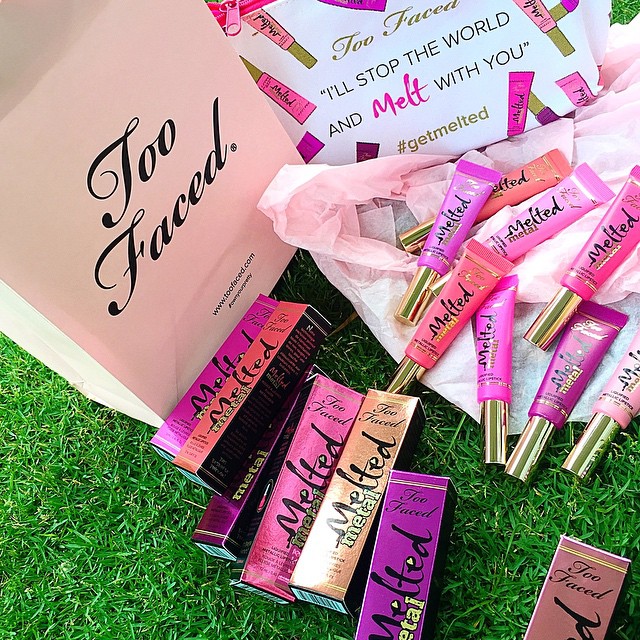This detailed photograph features an assortment of cosmetics from the brand Too Faced, all arranged on a vibrant green lawn. The centerpiece is a prominent pink bag with black lettering spelling out "Too Faced." Adjacent to the bag, various cosmetic tubes and boxes are scattered, showcasing bright and metallic hues of purples, oranges, and golds. These products, identified as "Melted" and "Melted Metal," feature colors ranging from light pink to dark violet. Some tubes sport gold caps, adding a touch of elegance. In the upper part of the image, two other bags are visible: one, a zip bag with the slogan "I'll stop the world and melt with you," accompanied by the hashtag #GetMelted, and the other bag simply displaying "Too Faced" along with the website www.toofaced.com. The overall presentation emphasizes the colorful and playful nature of the Too Faced brand amidst the lush green background.